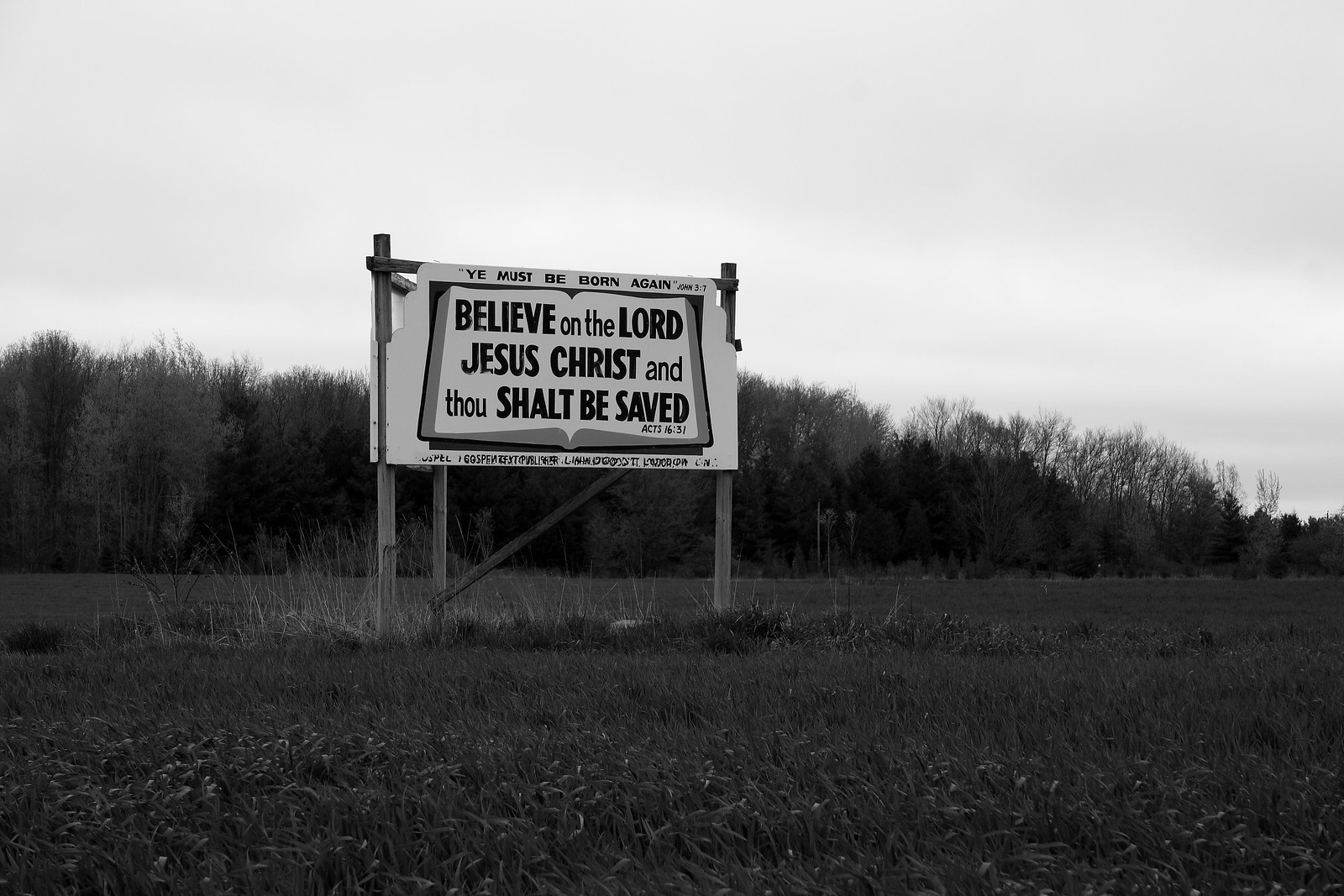This black and white image showcases a rustic wooden billboard, standing solitary in the midst of a wild, grassy field with trees lining the background. The billboard prominently features a large image of an open book, likely the Bible, with some depth effect that gives the impression you can see its side. Within the book's pages, bold text reads, "Believe on the Lord Jesus Christ, and thou shalt be saved," followed by the corresponding Bible verse reference. Above this central message, smaller text states, "You must be born again." There is additional writing at the bottom of the billboard, though it is too small to decipher. The wooden stand holding the billboard appears weathered and is missing its upper corners, adding to the rustic, unembellished aesthetic of the scene.